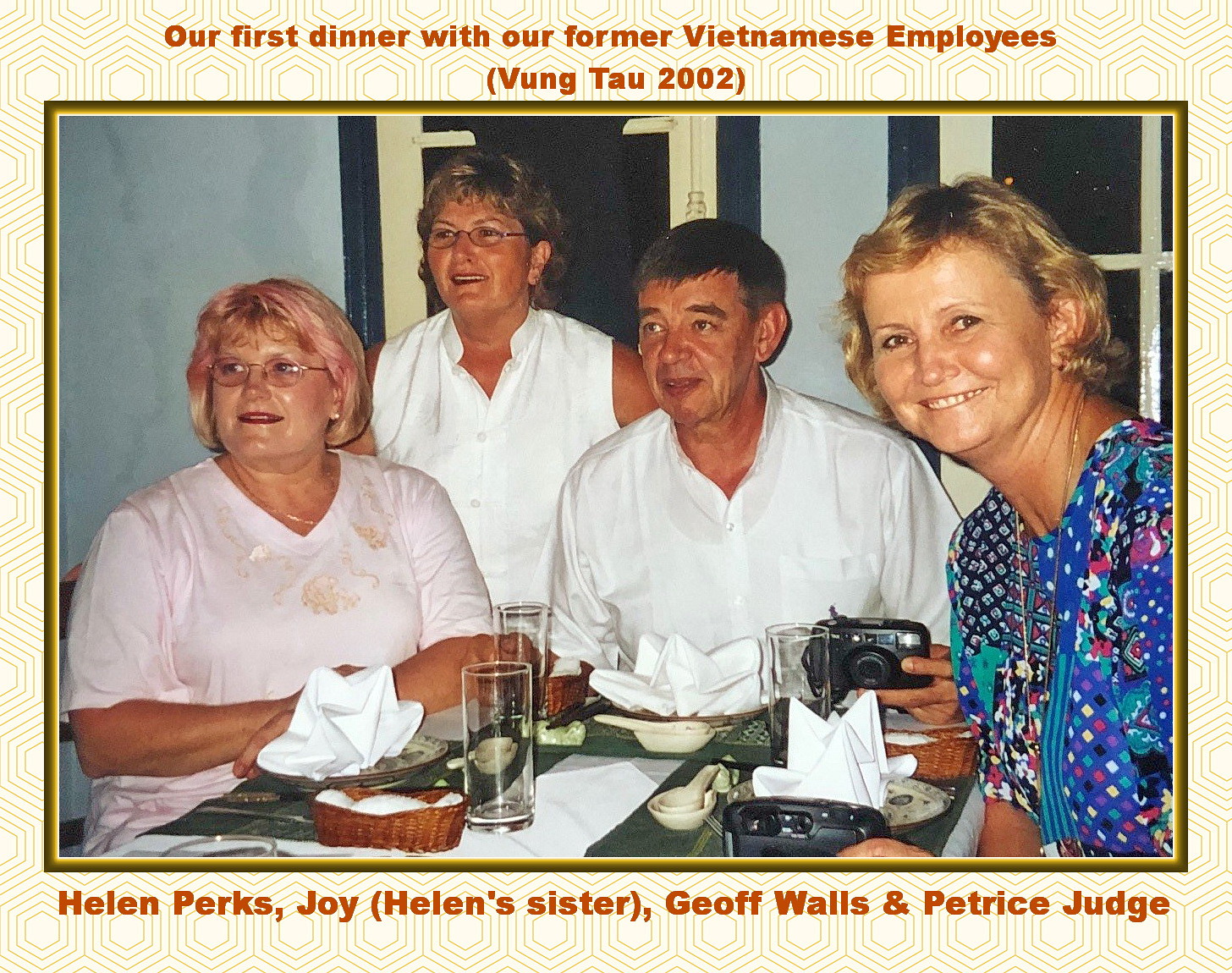The digitally framed photograph presents a scene from "our first dinner with our former Vietnamese employee Phuong Thao in 2002," as indicated by orange text above it. The hexagonal patterned frame in gold and white adds a geometric touch to the presentation. Below the photo, captions name the individuals as Helen Parks, Joy, Helen's sister, Jeff Walls, and Petrus Judge.

In the photograph itself, set within a darker gold frame, four individuals are seated and standing around a dining table adorned with serving ware, utensils, and empty plates, suggesting a recently finished meal. On the right side of the photo is Helen Parks, a Caucasian woman with blonde hair wearing a blue and multicolored patterned top, smiling at the camera. To her left is Jeff Walls, an Asian-looking man wearing a white shirt, holding a black, old-school camera in his left hand. Continuing leftwards, Joy is standing behind the table, wearing a white sleeveless button-down shirt and glasses, with brownish hair. On the far left, Petrus Judge, who has blonde hair with pink streaks and is wearing glasses and a pink top, is seated. The group radiates a sense of shared enjoyment and camaraderie post-dinner.